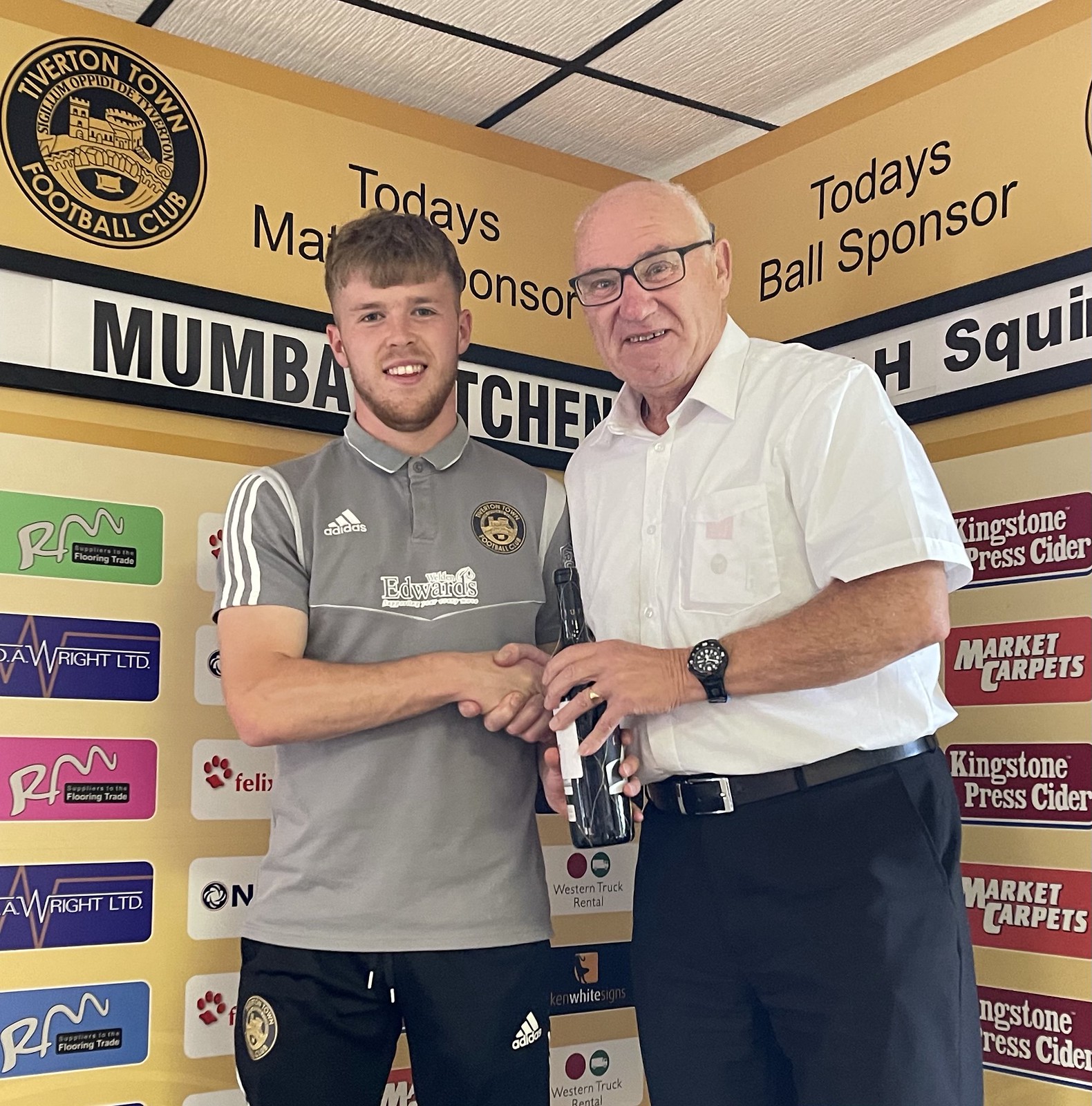The photograph depicts a moment of recognition within the walls of the Tibberton Town Football Club. In the center of the image, a young man, clad in a gray football jersey, warmly shakes hands with an older gentleman wearing a white shirt and black pants. Both individuals are smiling, suggesting the celebratory nature of the event. The elderly man holds a champagne bottle in his left hand, indicating a festive achievement, possibly an award or a victory.

Behind them, a yellow wall is adorned with various sponsor insignias and text, though much is partially obscured by the two figures. Prominently visible is the name "Tibberton Town Football Club" and mentions of "today's match sponsor" and "today's ball sponsor." Numerous sponsor logos, including Market Carpets and Kingstone Press Cider, are also scattered across the background. The setting appears to be a designated area for honoring players, perhaps on a dais where the club frequently acknowledges exceptional performances.